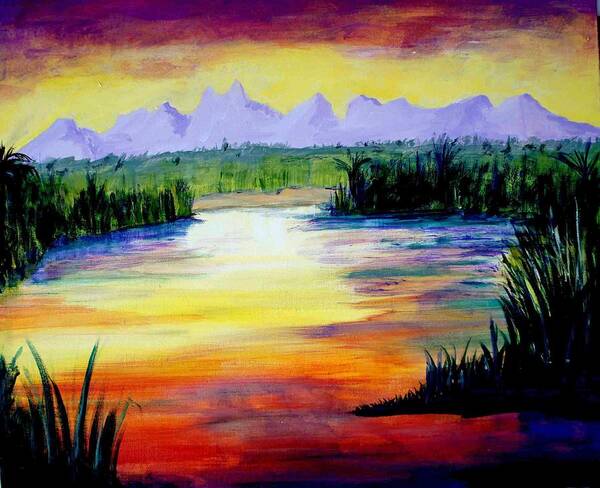This vibrant watercolor painting presents a vivid landscape dominated by a swampy body of water, taking up most of the image from the midpoint down. The water is a stunning array of horizontal streaks in reds, purples, yellows, oranges, blues, greens, and some touches of white, reflecting what appears to be a dramatic sunset. The sky above transitions from shades of yellow and orange to purples, casting a warm glow across the scene. The foreground offers an intimate perspective as if viewing from the position of someone standing in the water or on a canoe. Tall, green grasses with long, narrow leaves line the shore on either side of the water, some in shadow, adding depth to the scene. In the distance, a pastel purple mountain range stands majestically, completing the serene yet dynamic composition with an ethereal backdrop.